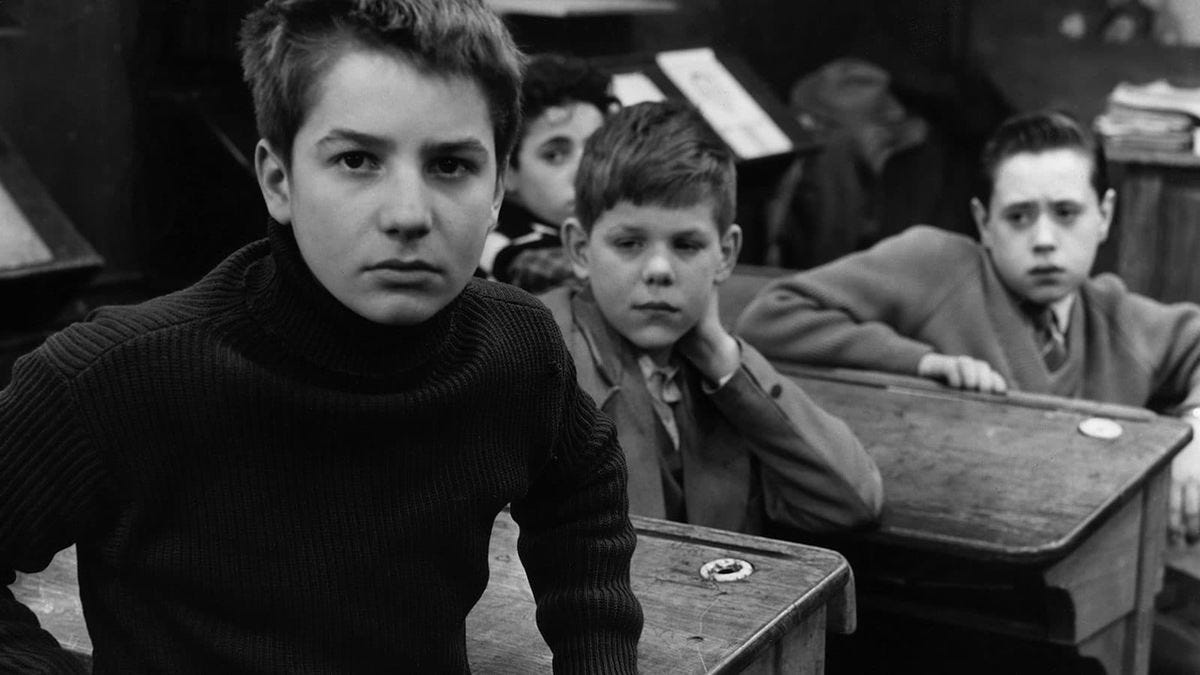In this evocative black-and-white photograph, likely taken several decades ago, a group of four boys, possibly aged between 8 and 12, are seated at old-fashioned wooden desks in what appears to be a school classroom, reminiscent of an English boarding school. The desks, equipped with inkwells, suggest a bygone era. 

The boy nearest to the camera, on the left, stands out due to his intense stare directly at the viewer, wearing a dark turtleneck sweater. His serious and pensive expression contrasts with the other boys, who also have dark hair and are dressed in long-sleeve shirts and sweaters, but are not making direct eye contact with the camera. 

Instead, these boys gaze off to the side, appearing somber and withdrawn. Behind the front boy, another child in a possibly suit jacket looks off to the side, while further back, a third boy wears a sweater layered over a tie and collared shirt. In the blurred background, hints of classroom supplies like books and stands are visible, adding context to the scholarly setting. The photograph captures a poignant, introspective moment from a bygone educational era.